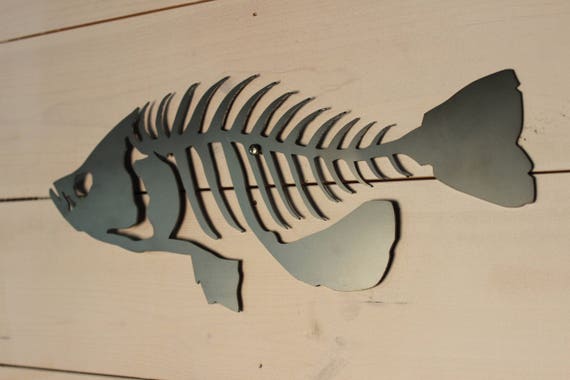This is a detailed color photograph in landscape orientation, capturing a piece of wall art in a residential setting. The background consists of beige, horizontal wooden planks, suggesting the siding of a house. Mounted on this wall is a decorative fish skeleton made of dark bronze metal, which appears slightly reflective with a metallic sheen in certain lighting. The fish skeleton is artistically crafted to resemble a realistic exoskeleton, with intricate details including the outlined face, eye hole near the mouth, vertebrae, and fins extending from the central spine. The head and tail are prominently outlined, and the skeleton tapers toward the tail, which is angled towards the right side of the image, giving an impression of movement to the left. Overall, the artistic style of the fish sculpture is representational realism, capturing the essence of a stripped fish in a lifelike manner.